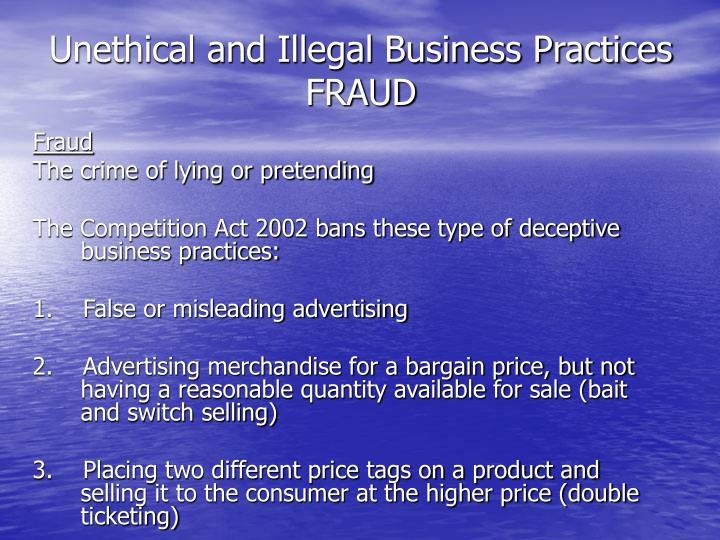The image is an informational slide with a blue background featuring an image of water at the bottom and sky with clouds at the top, suggesting it might have been created for a PowerPoint presentation or a similar format. The main text, in white letters, is clearly visible against this background. 

At the top, the title "Unethical and Illegal Business Practices: Fraud" is prominently displayed. Below the title, the term "Fraud" is underlined and defined as "the crime of lying or pretending." This is followed by a reference to the Competition Act of 2002, which bans deceptive business practices. 

The slide lists three specific types of fraudulent business practices:
1. **False or misleading advertising**
2. **Advertising merchandise for a bargain price, but not having a reasonable quantity available for sale** (noted as "bait and switch selling" in parentheses)
3. **Placing two different price tags on a product and selling it to the consumer at the higher price** (noted as "double ticketing" in parentheses)

This comprehensive overview aims to inform about various unethical and illegal business activities related to fraud, as detailed under the Competition Act of 2002.